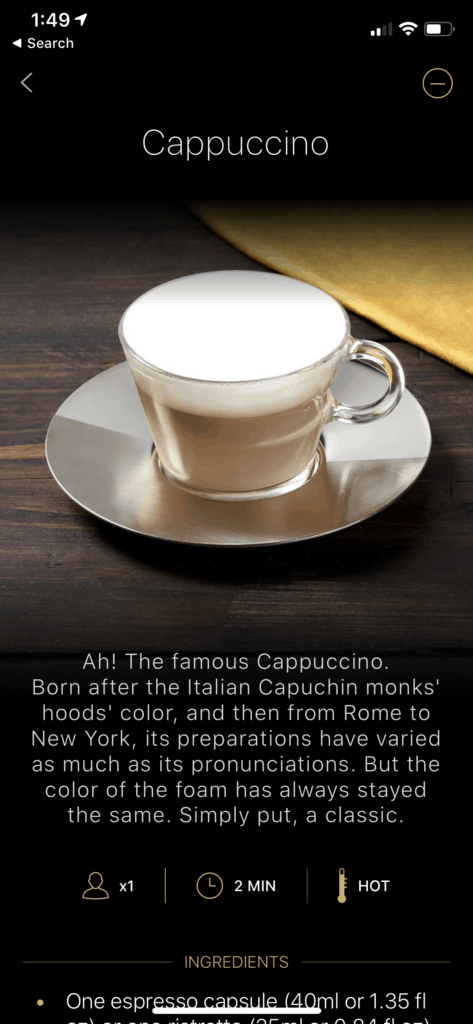The image captures the screen of someone's phone. At the top of the screen, the time is displayed as 1:49. To the right, there is a search icon followed by an arrow, and a circular icon with a minus sign inside. The connectivity status and signal bars are visible, showing about two-thirds battery life remaining. The background of the screen is predominantly black. 

In the center of the image, there is a visually appealing cup of cappuccino. The word "cappuccino" is prominently displayed in white lettering at the top against the black background. The setting features a wooden table or counter with a deep dark wood grain texture. Resting on the table is a clear saucer, upon which a clear glass cup is placed.

The cappuccino inside the cup is invitingly layered, with a rich brown, chocolatey coffee at the bottom and a creamy, fluffy white foam on top. The cup is equipped with a clear handle for easy holding. Below the image of the cappuccino, a paragraph reads: "Ah, the famous cappuccino, born after the Italian Capunchi monks' hoods color. From Rome to New York, its preparations have varied as much as its pronunciations, but the color of the foam has always stayed the same. Simply put, a classic."